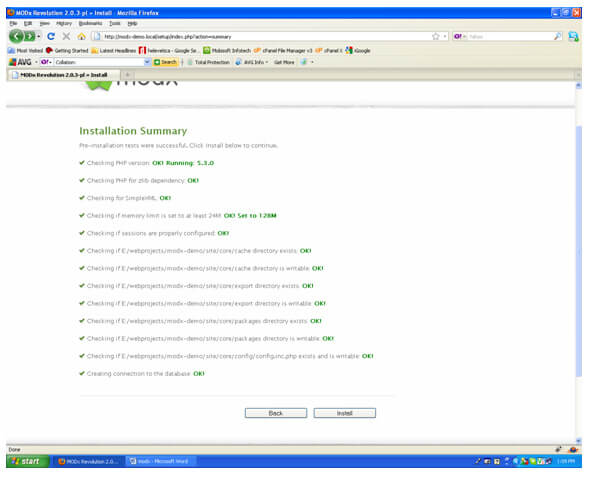The image displays a website with a navigation bar at the top, featuring various elements. On the left side, there's a green circular button with a white leftward arrow, while on the right side, there's a green square button with a white rightward arrow. These buttons possibly function as back and forward navigation controls. The navigation bar also includes a refresh button, a home icon, and a star icon, all arranged next to the website address bar. 

Adjacent to the address bar, there is a magnifying glass icon next to a search box. Below the navigation bar, the main content area contains an "Installation Summary" heading with a list of items. Each item in the list is followed by gray text and adorned with green checkmarks, indicating completion. To the right of this content area is a blue scroll bar, allowing users to navigate through the page content.

At the bottom of the page, there are two light gray rectangular buttons, labeled "Back" and "Install" in black text, suggesting options to either return to a previous step or proceed with installation.